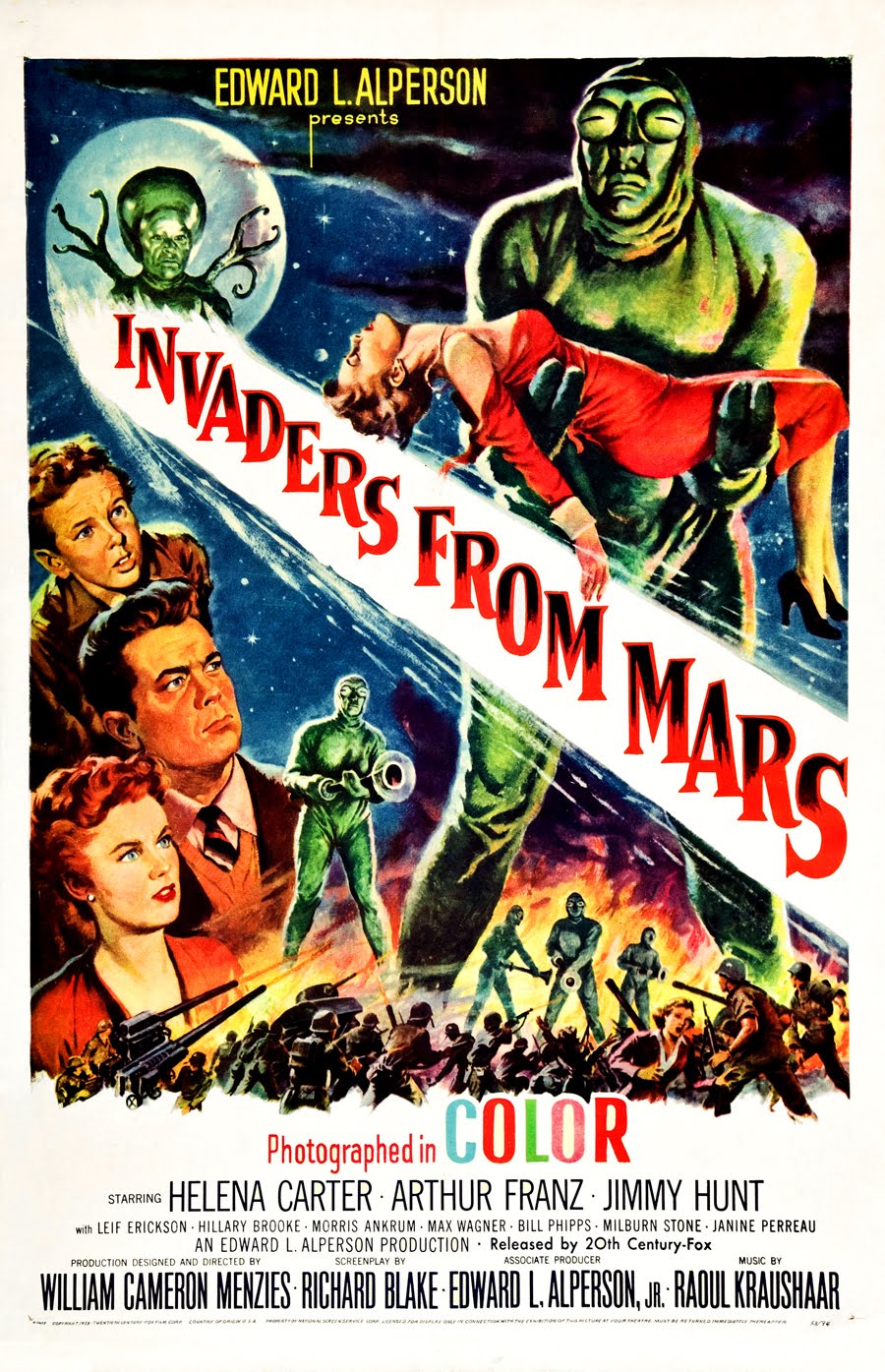This vintage movie poster for "Invaders from Mars," directed by Edward L. Alperson and released by 20th Century Fox, hails from the 1950s-60s era. Dominated by vivid yet limited colors, the poster prominently features the film title written diagonally in bold black and red letters, surrounded by a white strip to enhance visibility. Above the word "Invaders," a circular moon-like shape looms, adding to the extraterrestrial theme. 

The right side of the poster is taken up by a green-skinned, humanoid alien, complete with tendrils extending from its shoulders. This imposing figure clutches an unconscious woman with reddish hair, dressed in a knee-length red dress with long sleeves and white cuffs, and wearing black high-heeled shoes. The alien's hands appear gloved with only two fingers visible, emphasizing its otherworldly nature.

On the lower left side of the poster stands a small family—a man, woman, and child—gazing upward in fear. The woman has red hair and blue eyes, the man has dark, swept-back hair, and the child wears a brown shirt with brown hair. Nearby, another green alien brandishes a weapon, adding to the sense of imminent danger. In the background, a night sky stretches across the scene. 

Below the large alien, three smaller aliens appear with soldiers and tanks positioned underneath, aiming their weapons. A woman is seen fleeing among the smaller, fading images. The text at the bottom of the poster declares the film is "photographed in color," with the word "color" distinctively printed in various hues, and notable stars listed, including Helena Carter, Arthur Franz, and Jimmy Hunt. The comprehensive credits culminate in the 20th Century Fox logo, marking this historical film artifact.